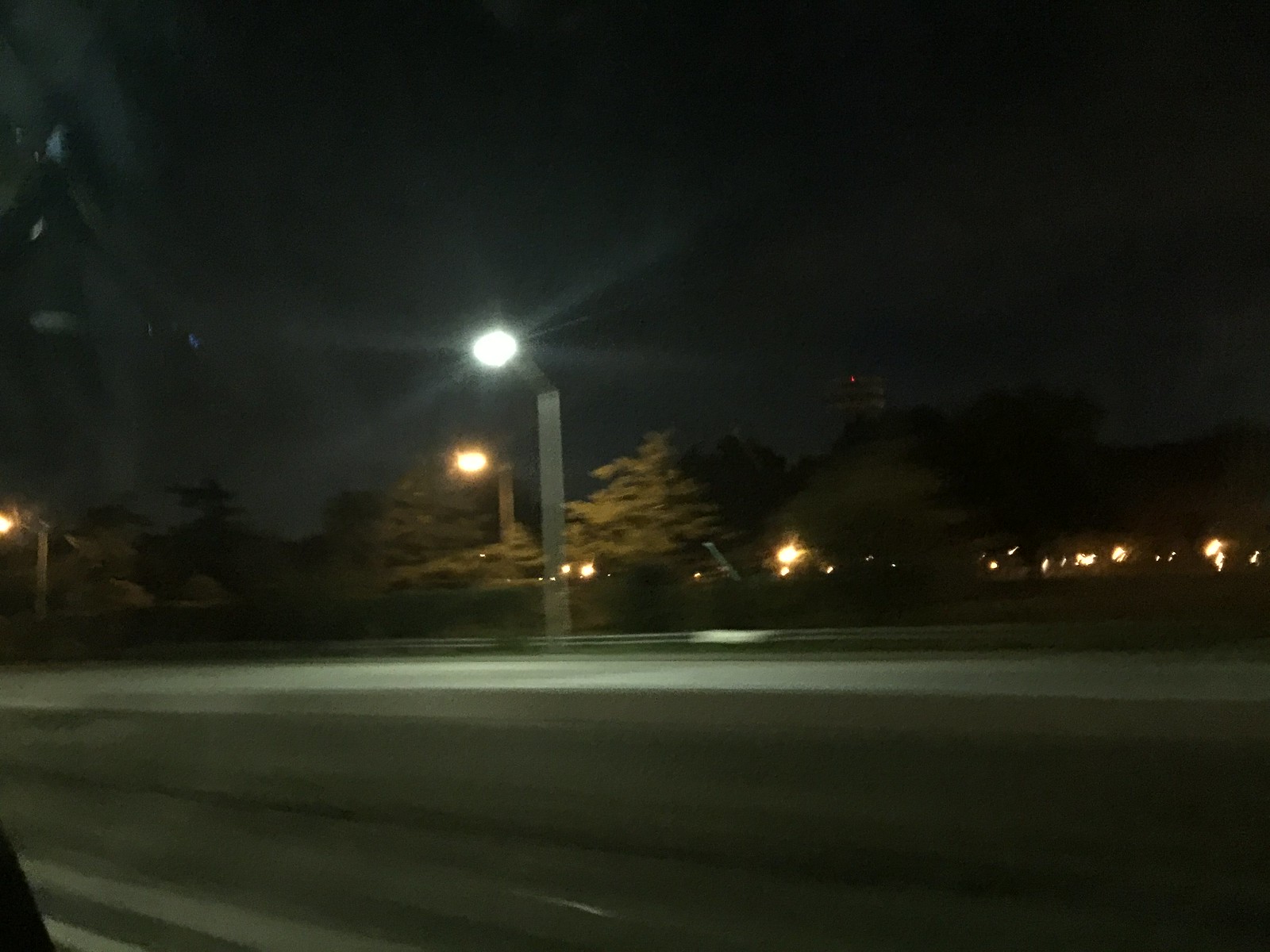A nighttime scene captured from the passenger seat of a moving vehicle shows a blurry landscape rushing by. The image, taken through the closed window of the car, features a few illuminated streetlights that cast a faint glow upon dark, empty pavement in the foreground. In the background, shadowy trees fade into the darkness of the night, interspersed with small points of light that may be emanating from nearby residential homes. The slight glare in the upper left-hand corner of the image, likely from the window, adds to the sense of motion and gives the photograph an ethereal quality.